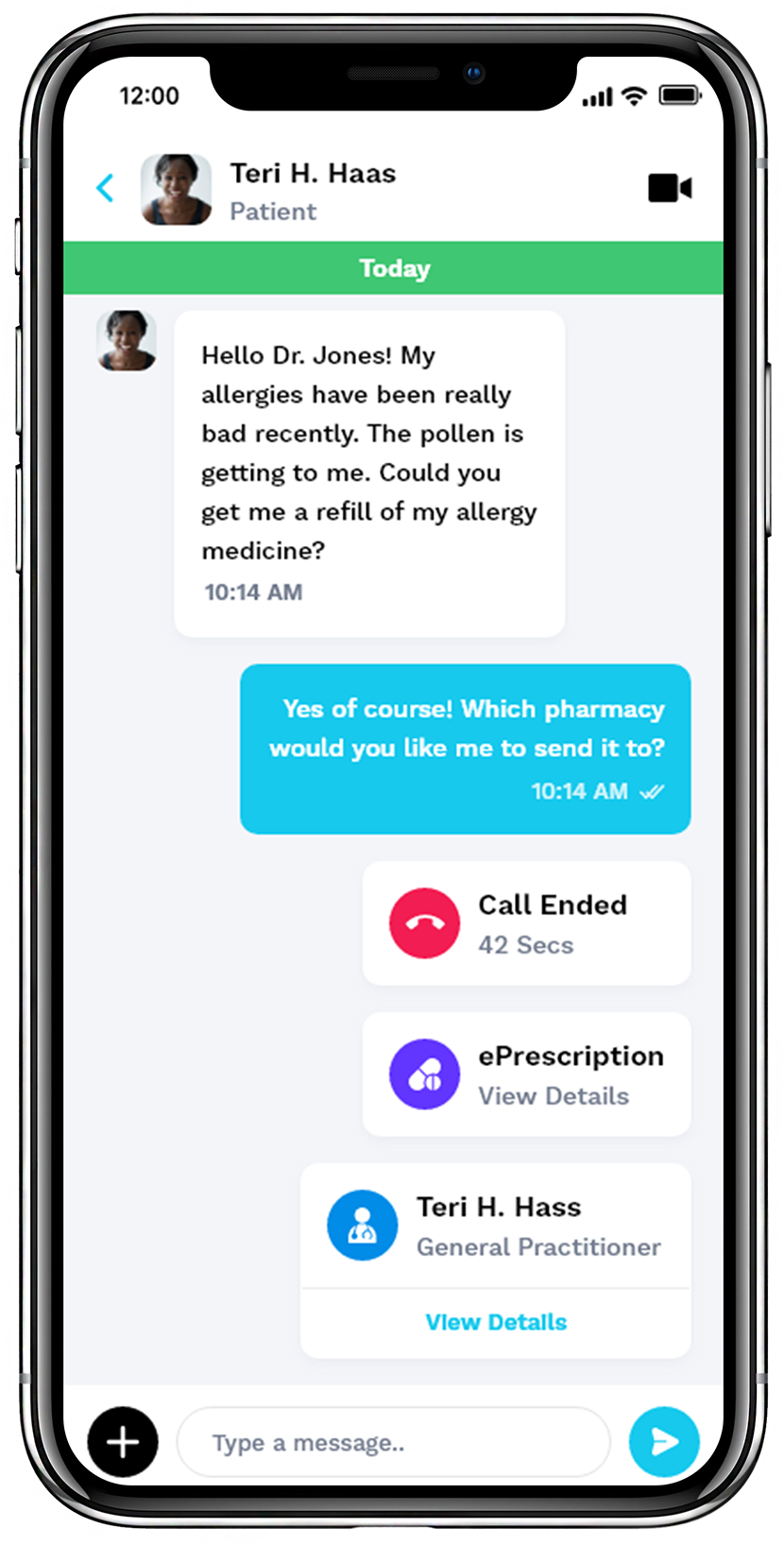The image is a detailed mock-up of an iPhone displaying a conversation between a patient and a doctor through a chat interface. The phone features a sleek metal frame and a distinct bevel around the screen. On the screen, we see a conversation between Terry H. Haas and Dr. Jones. 

On the left side of the conversation panel, there is a small photograph of Terry H. Haas, the patient, followed by a camera icon on the right. A green bar at the top indicates "Today." In the chat window, Terry initiates the conversation at 10:14 AM, with a message: "Hello, Dr. Jones! My allergy has been really bad recently. The pollen is getting to me. Could you get me a refill of my allergy medicine?" Dr. Jones responds promptly with, "Yes, of course. Which pharmacy would you like me to send it to?" also at 10:14 AM.

Below this conversation, there is a red circle with a phone icon and the text "Call ended 42 seconds." Below, there's an icon of pills labeled "E-Prescription" with a "View Details" option.

Further down the screen, another user icon is displayed with the name "Terry H. Haas, General Practitioner," followed by a "View Details" link in blue, which seems to be a mix-up since Terry Haas is the patient. The interface includes a black circle in the bottom left with a '+' sign for adding new information and a "Send" button next to a message input field.

This meticulously detailed mock-up highlights the streamlined functionality of a telehealth app, showcasing effective communication between patient and doctor, along with convenience features like e-prescriptions and messaging.